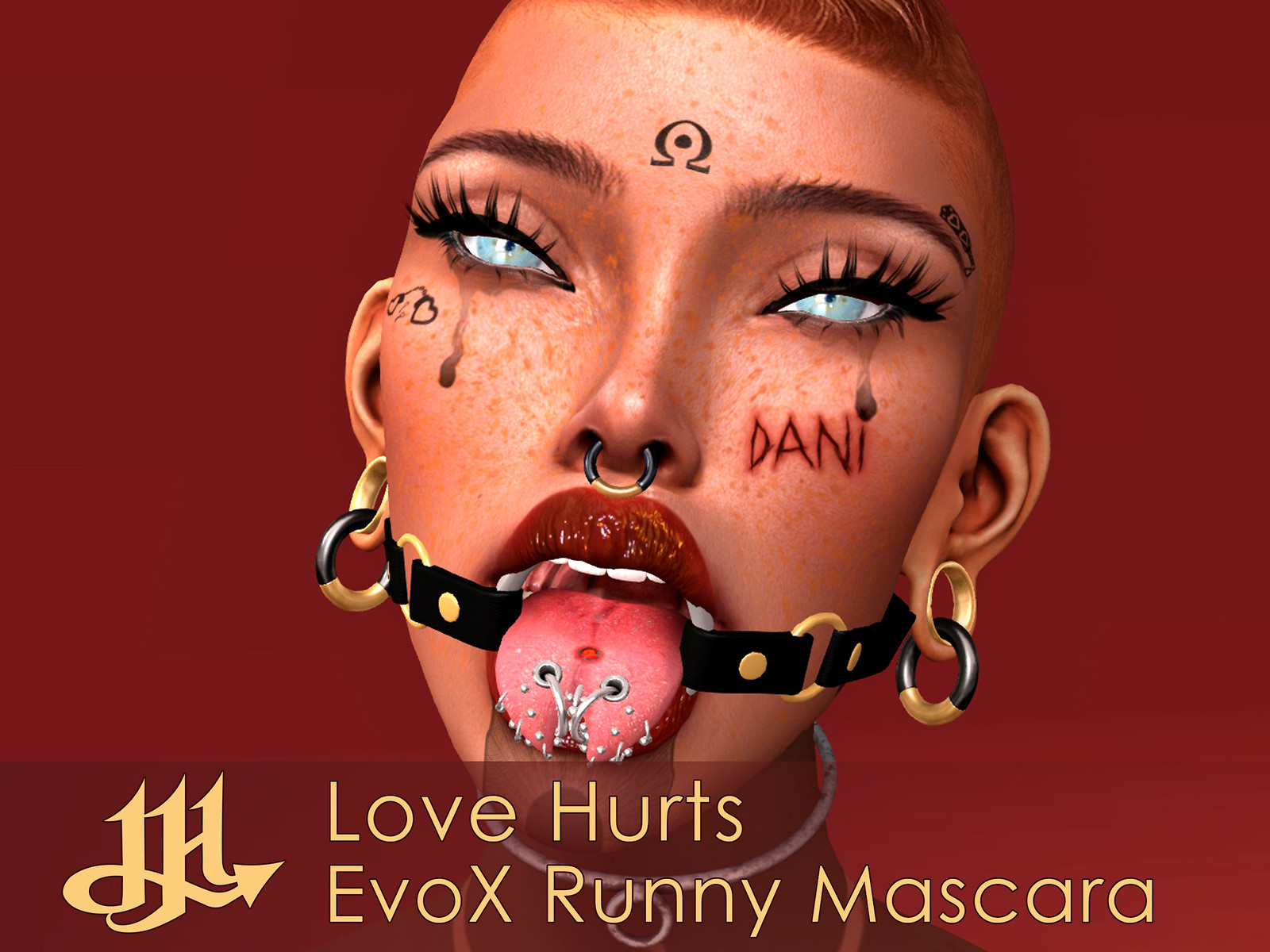The image depicts a striking and unconventional piece of art set against a deep red or maroon background, featuring a woman's face with very short, reddish-brown hair and prominent eyebrows. Her eyes are striking blue, accented by extraordinarily long eyelashes, and she has black mascara tears streaming from each eye. Below and to the left of the main image, yellow text reads "Love Hurts, EVOX, Runny Mascara," next to a Love Hurts symbol. The woman's face has a tattoo on her left cheek that spells "D-A-N-I" in red, accompanied by two teardrop tattoos. She wears two gold hoop earrings in each earlobe, with additional blue, green, and gold earrings hooked into the second hoops, causing her earlobes to stretch visibly. A leather strap, which seems to be connected to the bottom earrings, crosses her open mouth and sits under her tongue, exposing multiple piercings with dots indicating additional smaller piercings. Her lips are very red, and her tongue, which is equally vivid, is pierced multiple times. The woman's neck features a white necklace with a central white ring. The overall composition, combined with the intricate details of the piercings, tattoos, and accessories, creates a visually intense and evocative depiction of the phrase "Love Hurts."